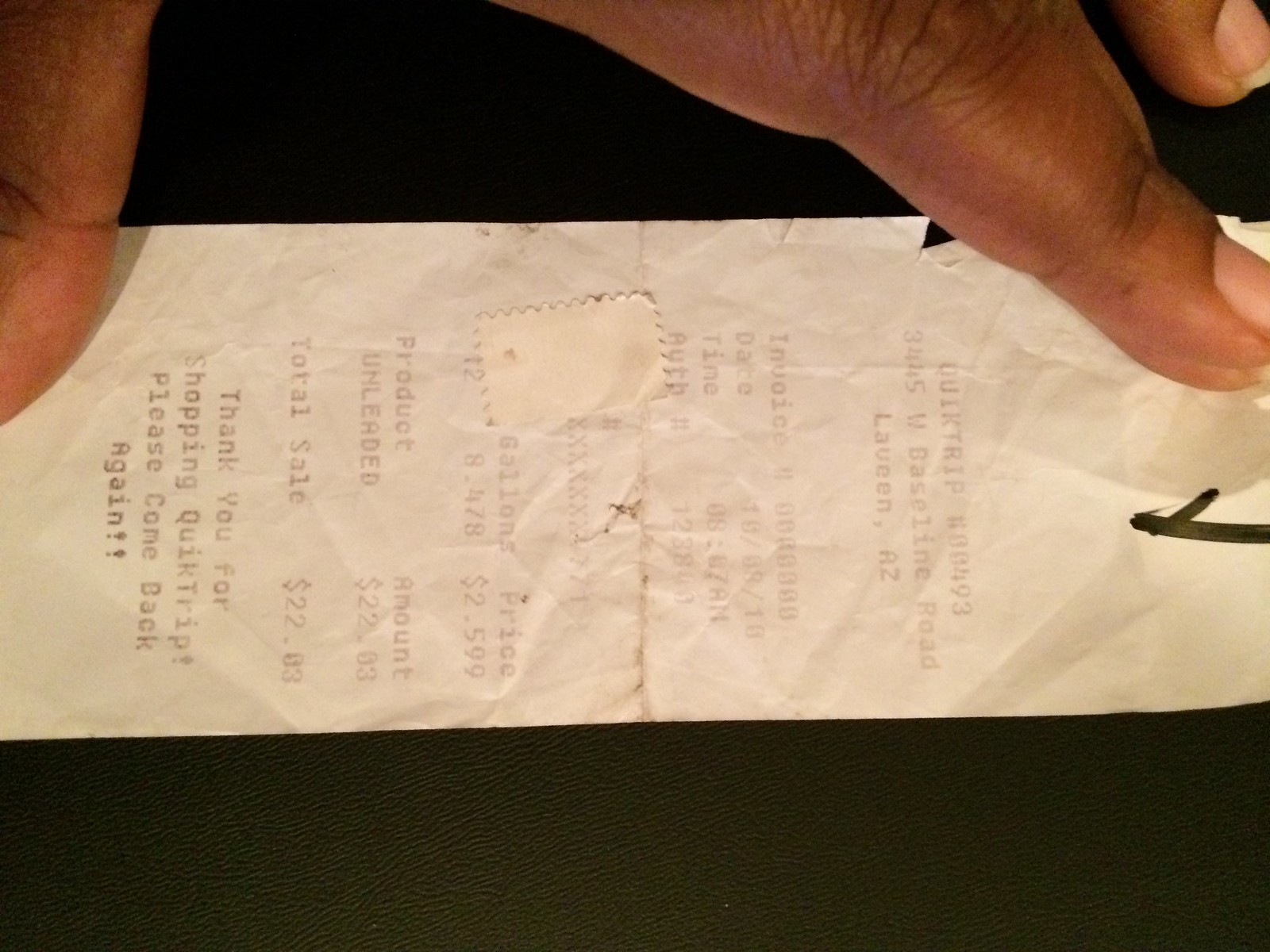A side-angle view of a receipt is held down on a black table by a person's hand. The receipt is positioned horizontally with the top of the receipt facing right and the bottom facing left. The person's thumb secures the bottom of the receipt on the left side, while the index finger holds down the top-left corner from the photo's perspective, revealing a part of their unpainted, slightly yellow middle fingernail. The receipt displays the store name "Quick Trip" at the top, although the remaining text is largely illegible. A small piece of fabric tape is attached to the left edge of the receipt. Additionally, a marker swipe is evident near the center top of the receipt. Towards the bottom, the receipt clearly displays "Total Sale 2203," and at the very bottom center, it reads, "Thank You for Shopping Quick Trip Please Come Back Again."